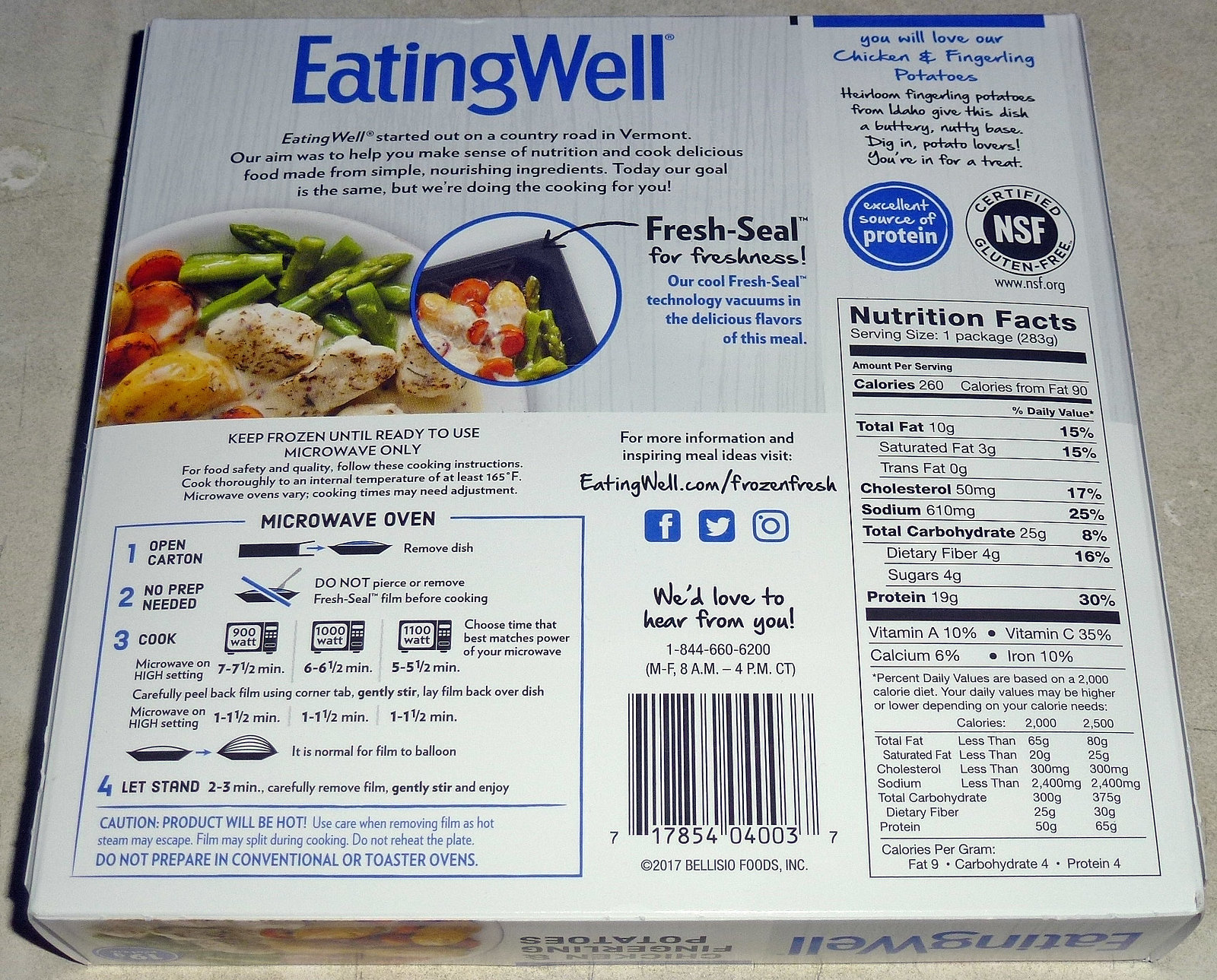Caption: 

The back of this frozen food box, set against a light gray or white background, features comprehensive branding and information aimed at appealing to health-conscious consumers. At the top, the phrase "Eating Well" is prominently displayed in blue, followed by a heartfelt origin story that begins, "Eating Well started out on a country road in Vermont." The text explains the company's mission to help consumers understand nutrition and enjoy delicious, simple, and nourishing meals, now conveniently pre-cooked. 

Below this narrative, a photograph showcases a delectable plate of chicken, asparagus, potatoes, and vibrant orange carrots, emphasizing the visual appeal of the meal inside. A notable "Fresh Seal for freshness" highlights the company's innovative vacuum-seal technology designed to lock in the meal's flavors. 

On the top right, the box promotes their "Chicken and Fingerling Potatoes" dish, adding that the heirloom fingerling potatoes from Idaho create a "buttery, nutty base," and invites potato lovers to indulge. Adjacent to this, a circle states "Excellent Source of Protein," and an oval verifies the meal as "Certified NSF Gluten-Free."

The box also includes detailed cooking directions for microwave preparation, outlined in four clear steps. Additionally, customer engagement is encouraged with the phrase "We'd love to hear from you," accompanied by a phone number. On the right side is a comprehensive nutrition facts panel, providing all the dietary details a consumer might need.